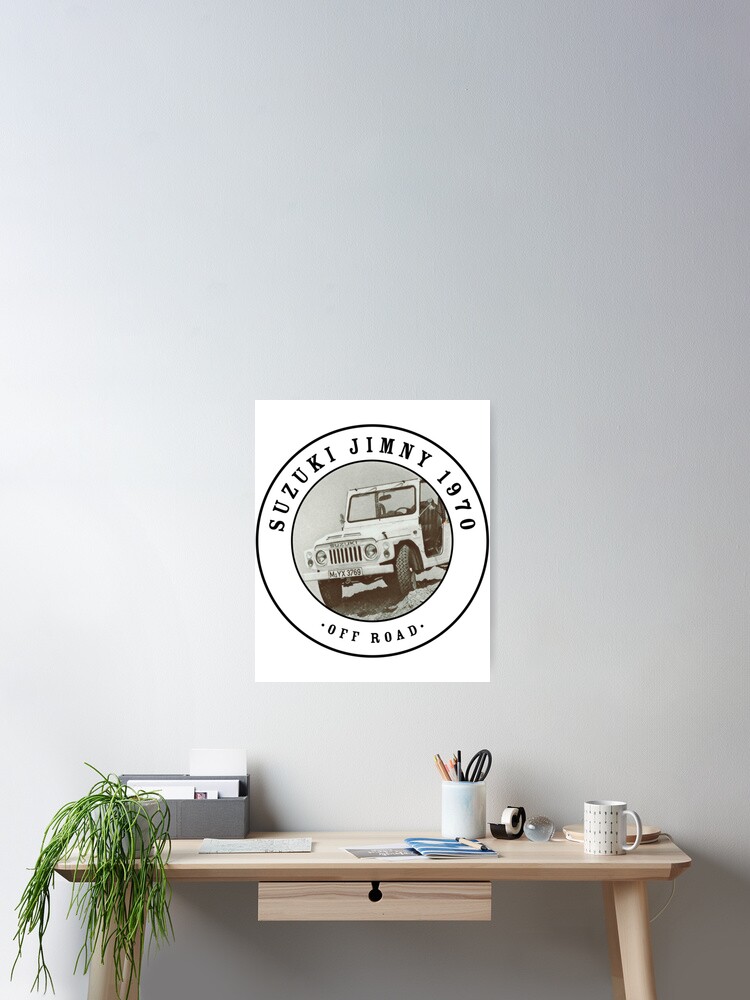The image depicts a minimalistic room with a light tan, possibly birch, wooden desk positioned against a plain white wall. The desk features a central drawer with a distinct keyhole-style cutout. On the desk, there is an assortment of items: a green plant with long vines, a gray file organizer, a small white desk lamp with a flexible neck, a white mug adorned with a pattern of dots, a tape dispenser, and a cup holder containing pencils and scissors. Various papers are scattered across the desk. Above the desk, a white poster prominently displays a circular design with the text "Suzuki Jimny 1970 Off-Road," encircling a black-and-white photograph of a jeep. The overall setup exudes a modern and clean aesthetic, with the white wall casting subtle shadows to enhance the minimalistic vibe.